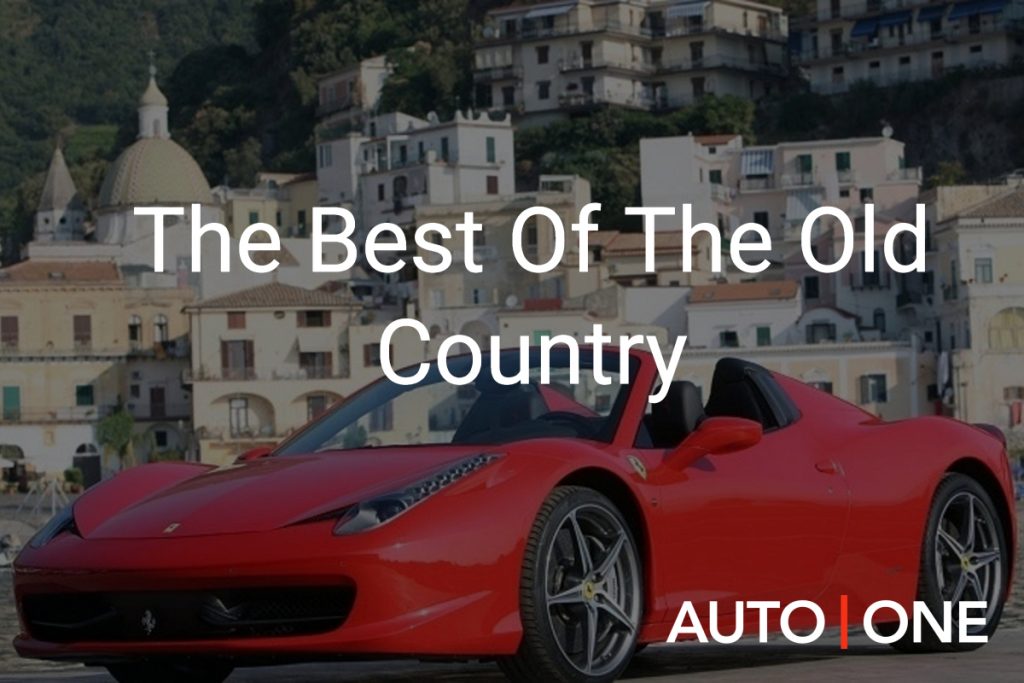The image features a sleek, futuristic red convertible sports car with no top, showcasing smooth lines and large black tires with silver rims. Prominently displayed on the grill is a horse logo. The picture includes text in the center reading "The Best of the Old Country," with "Auto One" in the bottom right corner. The background is a picturesque European town, characterized by white buildings and structures climbing up a hillside interspersed with greenery, evoking the charming architecture of places like Greece, Italy, and Spain, complete with both triangular and dome roofs.